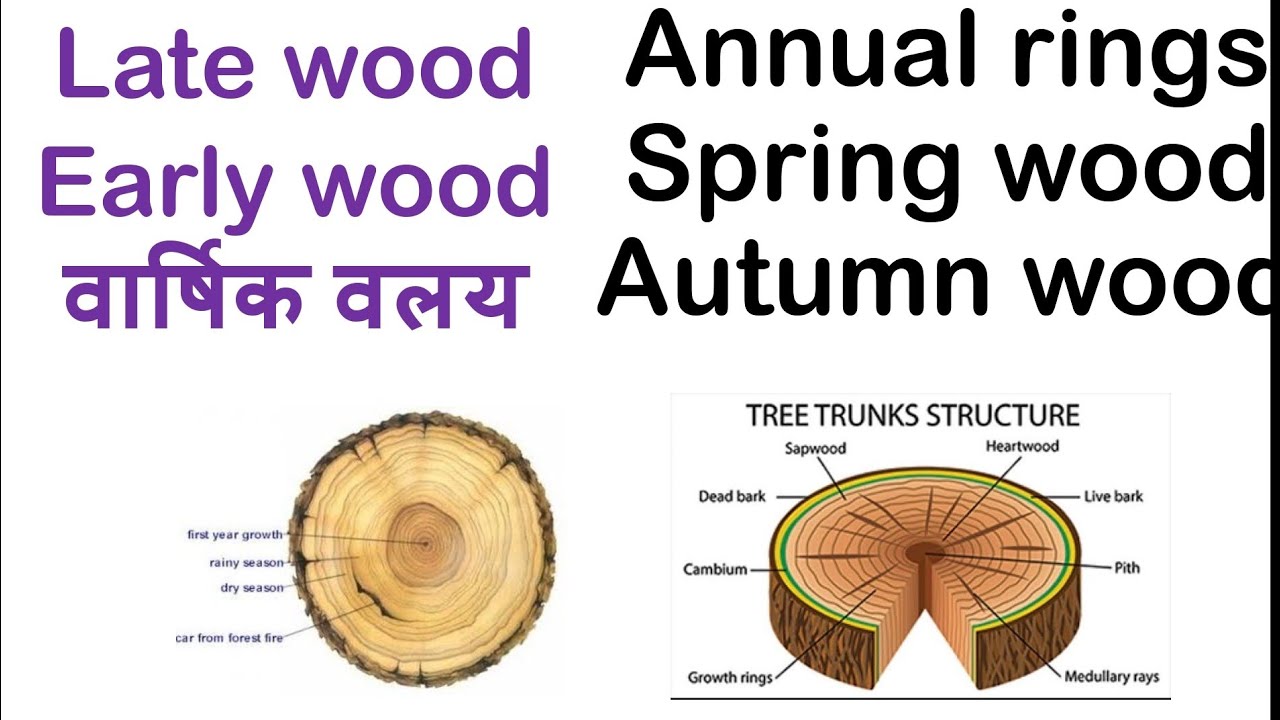The image displays a detailed view of different stages and structures of wood, set against a solid white background. On the left, there is a cross-section of a tree trunk showing the rings from an above angle, accompanied by labels: "first year growth," "rainy season," "dry season," and "scar from forest fire." Large text in purple labels the areas as "late wood" and "early wood." The right side provides a comprehensive diagram of a tree trunk's structure, labeling "annual rings," "spring wood," "autumn wood," and illustrating components such as "sapwood," "heartwood," "dead bark," "live bark," "cambium," "pith," and "medullary rays," with arrows pointing to each part. The visual elements elucidate the intricate details of wood growth and seasonal changes.